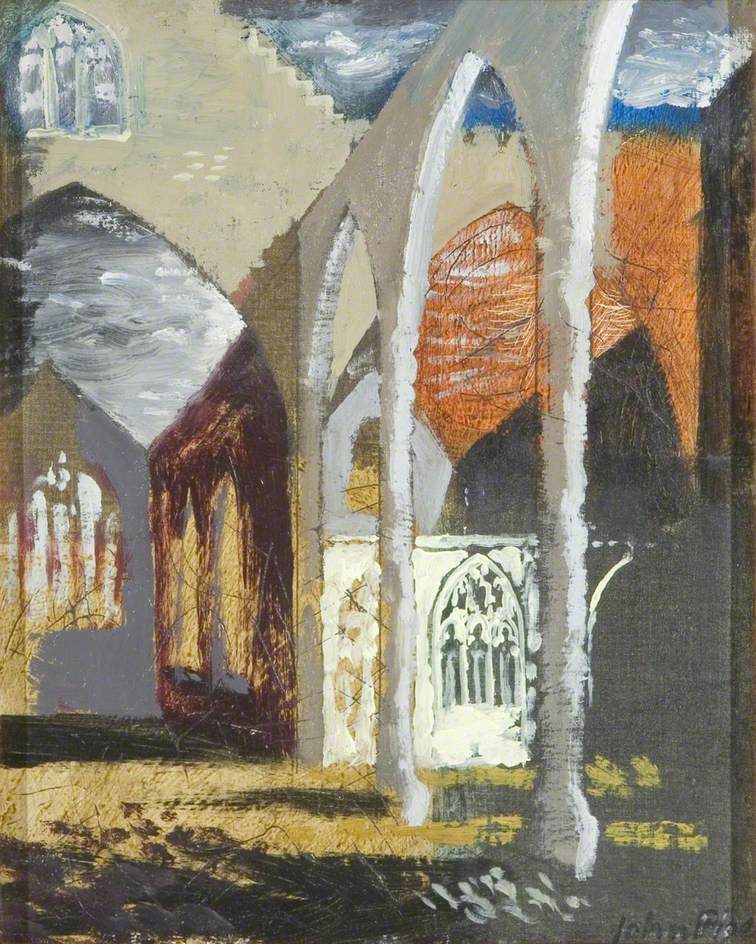This painting depicts a detailed architectural structure, rendered in watercolor with a somewhat old and smudgy appearance. On the right side, there's a prominent white section featuring a series of tall columns supporting arches that come to a dull point at the top. Below this section, through one of these archways, there's a display resembling a window with shadows or silhouettes of three people. In the bottom right corner, the artist's name, John, is visibly signed. The left side of the painting shows another entrance with a similarly shaped archway, topped by a gray roof and a light cream-colored wall that has hints of blue and purple, accented with gold. The scene is set against a backdrop of a sky that transitions from a bluish hue at the bottom to a mix of gray and white clouds above. There's a patch of light brown grass at the base, while the top right corner of the painting incorporates an orange hue blending into the sky.